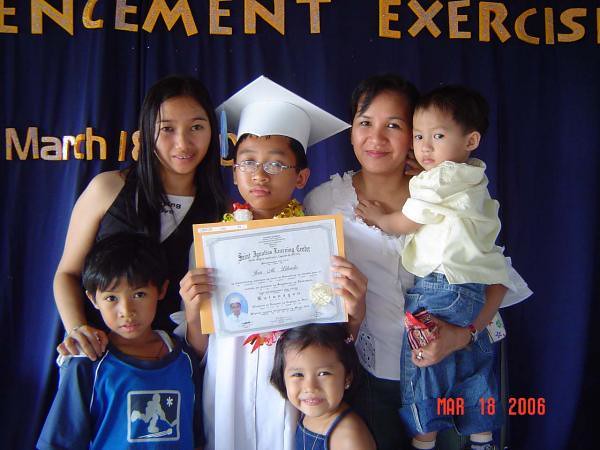In the photograph, a family is gathered in front of a dark blue curtain with partially visible block yellow text behind them, including the words "commencement exercise" and the date "March 18, 2006." Central to the image is a young boy wearing glasses and dressed in a white graduation cap and gown with a blue tassel. He proudly holds a diploma. Surrounding him are three other children: a girl dressed in black, a little boy in a blue shirt, and another smiling girl at his side. To the right stands a woman, possibly their mother, holding a baby. They all appear to be of Asian descent and are smiling directly at the camera, commemorating what seems to be a special graduation event.